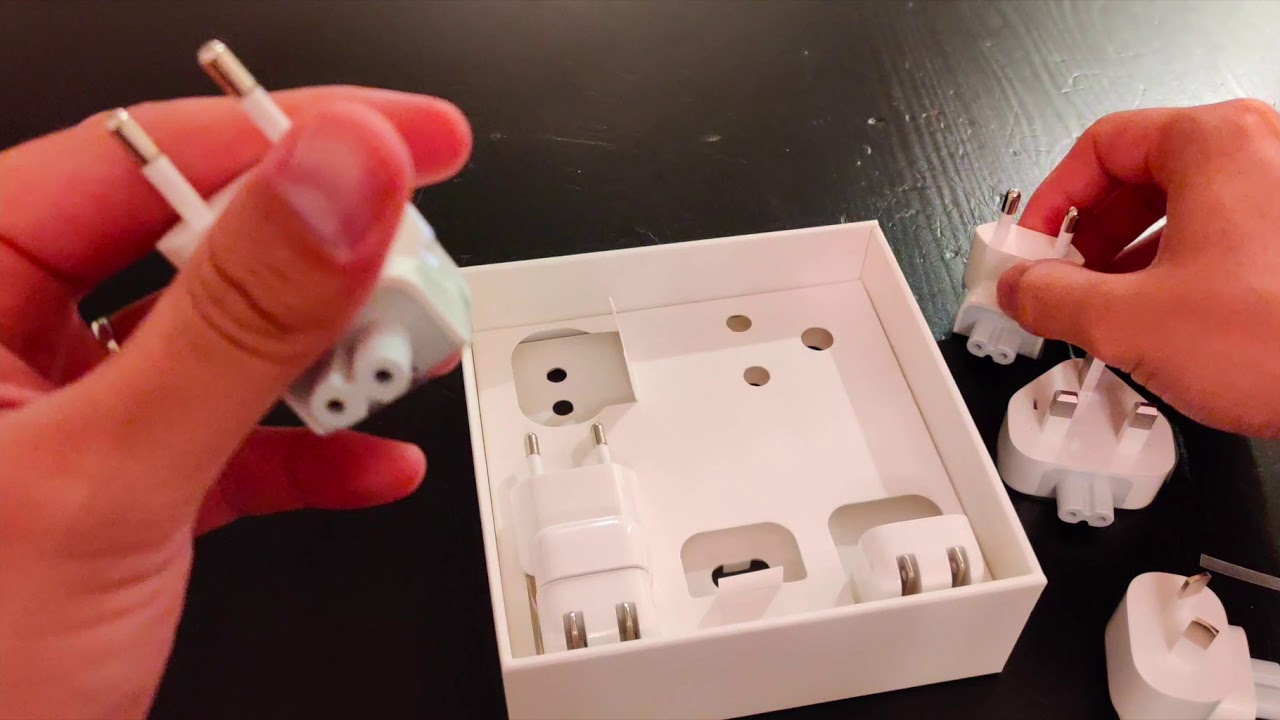The horizontally rectangular, full-color photograph, clearly staged indoors, features a dark brown wooden countertop devoid of any additional background. Positioned towards the upper right-hand corner, there is a subtle touch of light shining through. The image centers around a pair of Caucasian hands—one on the left and one on the right—each holding a white plastic plug with silver metallic prongs. In the middle of the composition is a white cardboard box segmented into multiple slots, containing various similar plug components. On the tabletop, particularly on the bottom right-hand side, lie additional plug pieces. The setting gives a sense of a potential unboxing or assembly event, possibly involving compatibility adapters for devices, as these white plugs with silver elements resemble those used in chargers, perhaps akin to MacBook chargers.